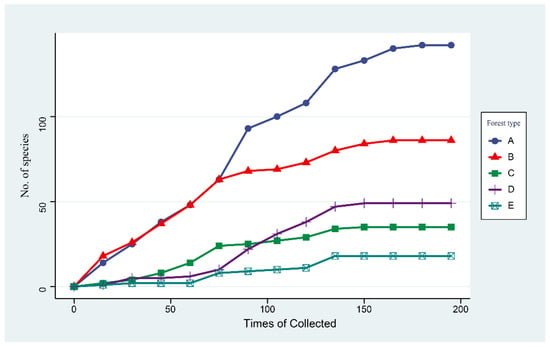The image displays a detailed chart on a light blue background, featuring a white rectangle containing five lines in different colors: blue, red, purple, green, and aqua. The left side of the chart is labeled as "Number of Species" with values at the top marking 100, marked midway at 50, and the baseline at 0. The bottom axis is labeled "Times Collected," with intervals marked from 0 to 200 in increments of 50. 

In the top right corner, there is a white rectangle outlined in black labeled "Forest Type," serving as a key for the colored lines: dark blue (A), red (B), green (C), purple (D), and aqua (E). The blue line rises sharply from 0 to over 100, the red line ascends to around 80, the purple line peaks around 50, the green line reaches up to 40, and the aqua line climbs to about 25. The chart details the number of species collected over varied times, corresponding to the different forest types represented by the color-coded lines.